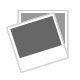This is a detailed photograph of a single pair of Sperry Top-Sider sneakers, presented in a portrait layout with the shoes arranged vertically against a white background. The image is taken from an overhead perspective, showcasing the navy blue canvas material of the shoes. Each shoe features light brown laces that are tied into knots at the top eyelets, creating a casual and stylish appearance. The brand "Sperry" is prominently displayed on the tongues, and inside the shoes, the insoles read "Sperry Top-Sider" in silver lettering. The shoes, which exhibit a low-top design and white side soles, appear to be in excellent condition, suggesting that they are either new or barely worn.